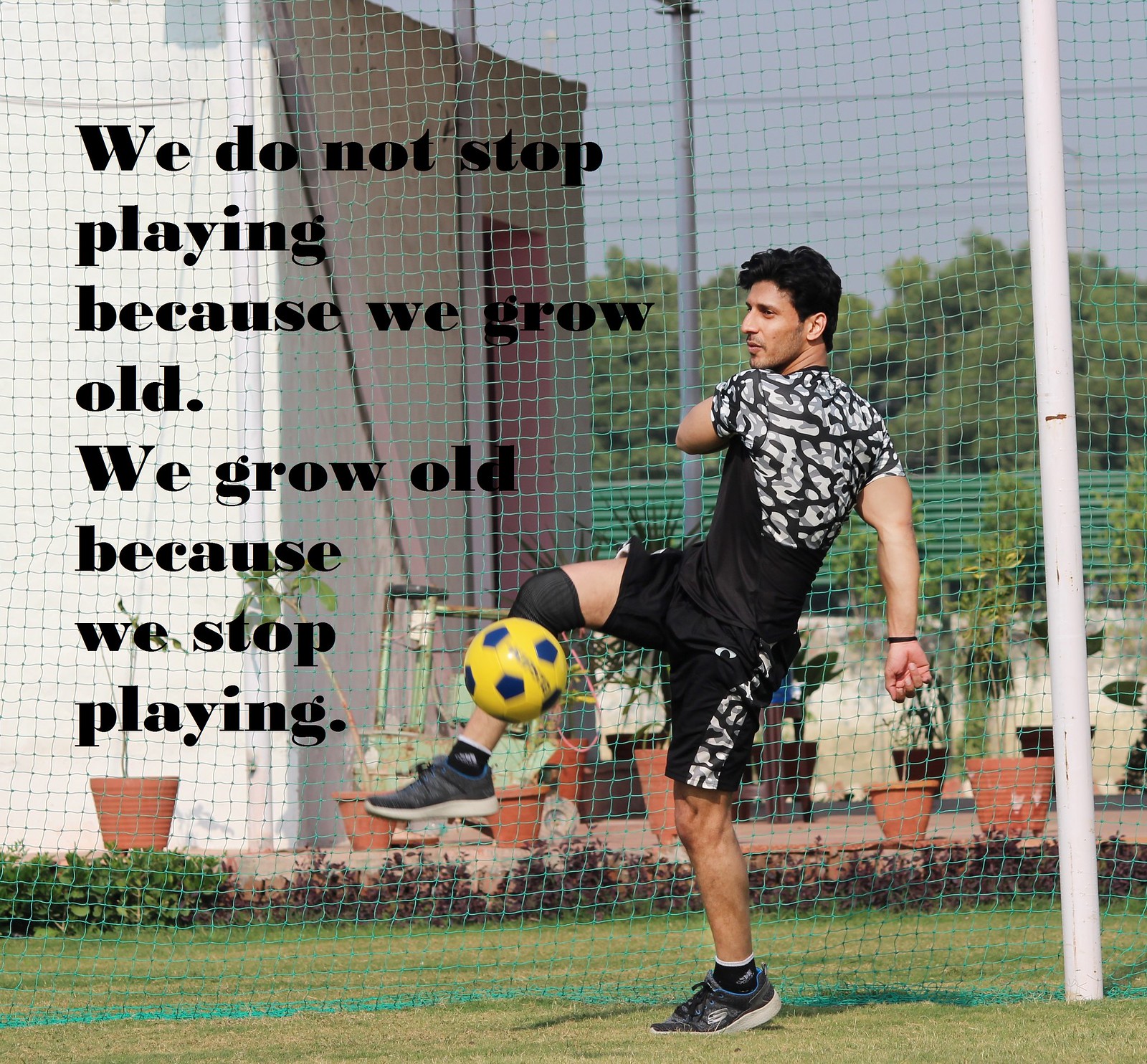The image depicts a soccer player in action, wearing a black and white uniform, including a shirt and shorts with a black and white stripe down the left side. He has a brace on his right knee, a knee pad ideally, and dark hair. The player is captured mid-kick, standing on his left leg with his right leg extended to kick a soccer ball, which is yellow with dark blue accents. His right arm is stretched towards the ground, while his left arm is bent behind him. He is positioned inside a goalie net with white posts and green netting, standing on a lush green grass surface. In the background, the net reveals an assortment of potted plants with green foliage in both terracotta and dark brown pots. Further behind, a green fence and trees can be seen. On the left side of the image, a motivational quote in black lettering reads, "We do not stop playing because we grow old. We grow old because we stop playing."